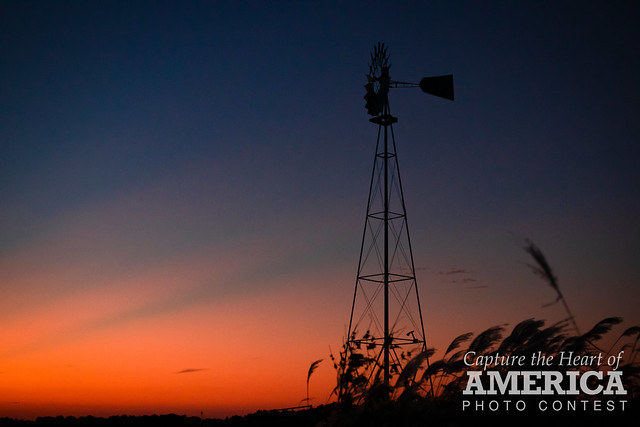This detailed square photograph captures a mesmerizing outdoor scene at either sunset or sunrise, evident from the gradient sky transitioning from a vivid orange in the lower left to a deep, almost black, blue towards the upper right corner. Dominating the image is an old-style metal windmill, positioned slightly right of center. The windmill features a disc-shaped impeller, oriented with its blades facing left, while its tail fin extends to the right. Beneath the windmill, one can spot wheat stalks and various forms of brush, possibly including pieces of tumbleweed, suggesting a windswept environment. Despite the ambiguity of its motion, the surrounding vegetation hints at a brisk wind. Adding a sense of contest excitement, the bottom right corner contains bold white text announcing "CAPTURE THE HEART OF AMERICA PHOTO CONTEST." Small clouds scatter across the sky, enhancing the picturesque quality of this compelling snapshot of rural America.